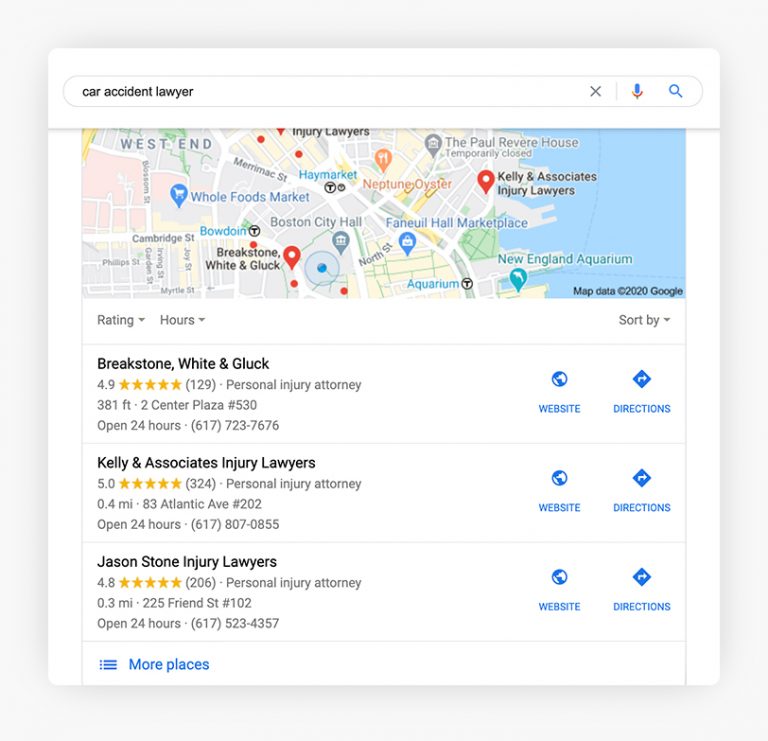The screen capture depicts an active search for a "car accident lawyer" conducted on a PC or laptop. At the top of the image, the search term "car accident lawyer" is visibly entered in the search bar, accompanied by a microphone and magnifying glass icon in the upper right corner. Beneath the search bar, a Google Maps section is displayed, focusing on the Boston, Massachusetts area, specifically highlighting landmarks such as Boston City Hall and Payonell Hall Marketplace.

The map features several marked locations: two red pins, a green pin, an orange pin, two gray pins, and two blue pins. Users can sort search results by "rating" and "hours," with additional filtering options accessible via a "sort by" button, all featuring drop-down arrows for further customization.

On the left side of the screen, three listings of personal injury attorneys appear:
1. **Breakstone, White, and Gluck** - This listing includes the description "personal injury attorney" and features icons for the website (globe) and directions (blue triangle with a white arrow) on the right.
2. **Kellyanne Associates** - Labeled as "injury lawyers, personal injury attorney," it retains the same website and directions icons on the right.
3. **Jason Stone Injury Lawyers** - Also identified as "personal injury attorney," with the same website and directions icons on the right.

All the listed attorneys have ratings ranging from 4.8 to 5 stars. At the bottom left corner of the screen, a "more places" option is available in blue, indicating additional search results or locations.